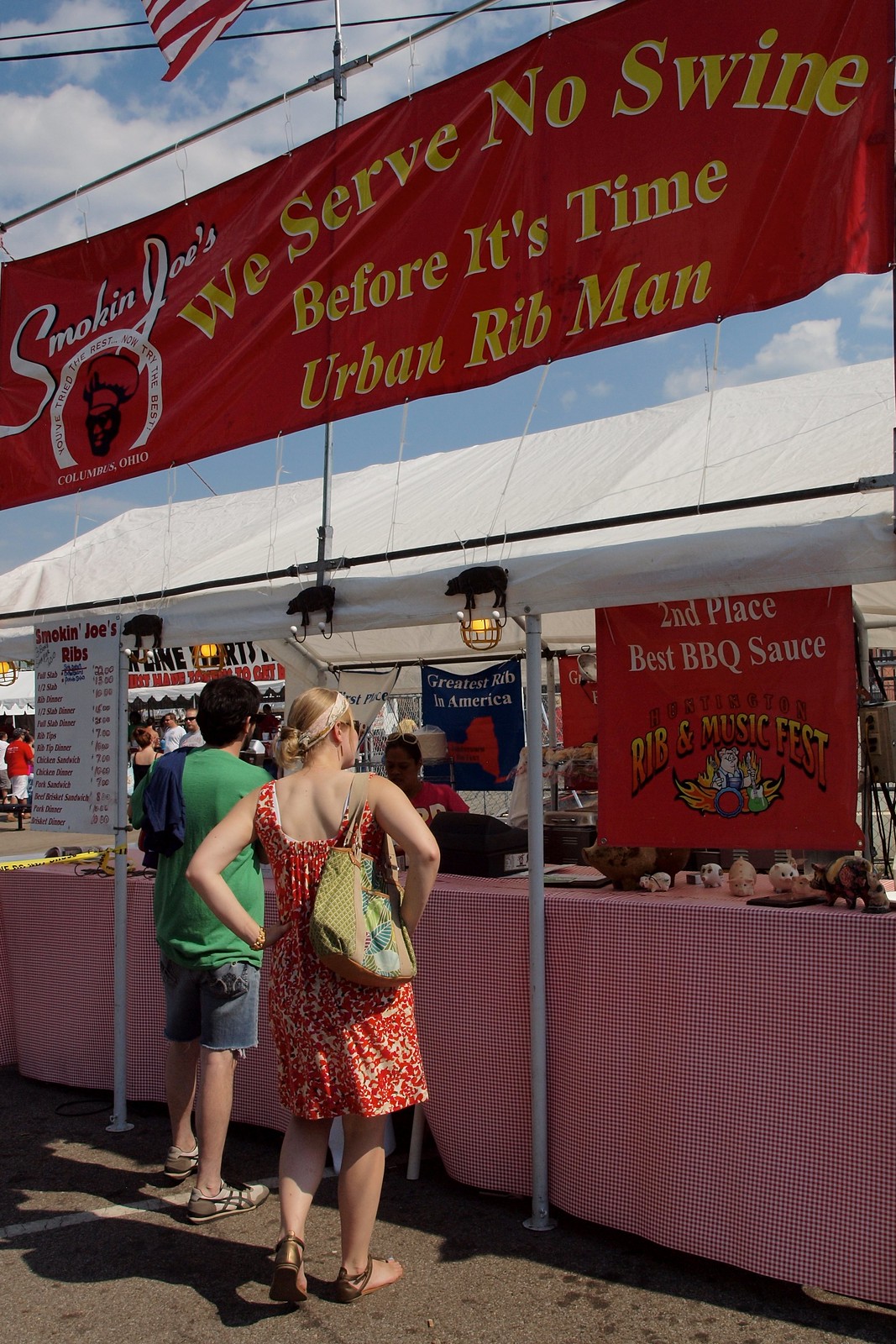In the midst of a bustling festival, an inviting rib tent named "Smokin' Joe's" stands proudly under a vivid blue sky dotted with a few clouds. The prominent red banner with bold white lettering announces "Smokin' Joe's," while a yellow script beneath it proclaims, "We Serve No Swine Before It's Time," followed by the moniker "Urban Rib Man." A smaller sign boasts their accolade: "Second Place Best Barbecue Sauce, Ribs and Music Fest." Positioned in front of the tent, a woman in a red polka dot dress with a bandana over her blonde hair stands next to a man wearing a green shirt and blue cut-off jean shorts, with a shirt casually draped over his shoulder. Both await their turn to order from the bustling food stand, where a team is busy cooking and selling their renowned ribs. The scene is complemented by the checkered red tablecloth of the counter, strewn with various trinkets, and a detailed price menu on one side. The background reveals more tents and festival-goers, adding to the lively atmosphere. Above it all, a barely visible American flag flutters, adding a touch of patriotic charm to this vibrant street food setting.